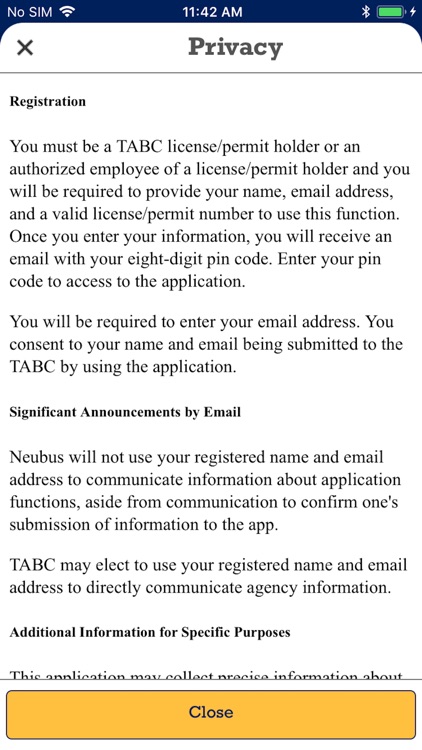This image is a detailed screenshot from a smartphone. At the very top, there's a dark blue border. Centered within this border, in white text, is the time displayed as "11:42 a.m." On the left corner, the text "No SIM" is shown in white, indicating the absence of a SIM card. Next to this text, there is a Wi-Fi icon, suggesting the device is using a Wi-Fi connection. On the right side of the top border, a green battery icon is displayed, indicating a fully charged battery, and beside it, there is a white Bluetooth icon.

The background of the screen is white. At the top center of this white background, the word "Privacy" is written in gray font. Immediately below this, there is a line separating the header from the main content. On the left side of the line, a small gray "X" is present, which likely serves as a button to close the page.

Beneath this section, on the left side, the text "Registration" is noticeable. This appears to be the beginning of a detailed explanation about the registration process for a specific account. The text informs that the user must be a TABC license/permit holder or an authorized employee of a license/permit holder. It states that the user will need to provide their name, email address, and a valid license/permit number to use the function. It further explains that after entering this information, the user will receive an email containing an eight-digit PIN code, which is needed to access the application.

At the very bottom of the screen, there is a gold-colored rectangle button. In the center of this button, "Close" is written in the same dark blue font, indicating that clicking this button will close the screen.